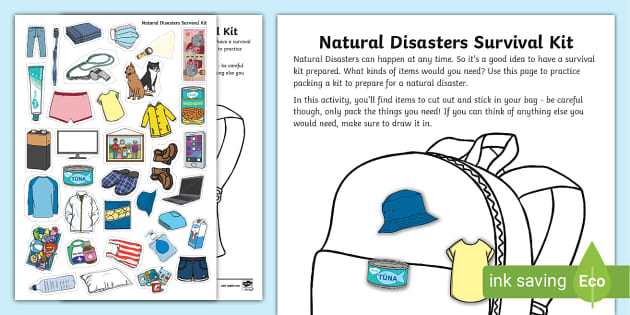This image appears to be an illustrative workbook page designed to educate children about preparing a Natural Disaster Survival Kit. In the upper right-hand corner, it prominently features the title "Natural Disaster Survival Kit." Below the title, the text reads, "Natural disasters can happen at any time, so it's a good idea to have a survival kit prepared. What kinds of items would you need? Use this page to practice packing a kit to prepare for a natural disaster. In this activity, you'll find items to cut out and stick in your bag. Be careful though, only pack the things you need. If you can think of anything else you would need, make sure to draw it in."

The right side of the page includes an illustration of a backpack, to which two stickers are already attached—a blue hat and a can of tuna fish. The lower right-hand corner indicates the page is "Ink Saving Eco." The left side of the image showcases a variety of stickers depicting items one might need in a survival kit. These items include canned goods, a cell phone, boots, slippers, hats, t-shirts, batteries, and other essential items. This engaging activity aims to help children understand and practice essential emergency preparedness skills by selecting and placing relevant stickers on the backpack illustration.